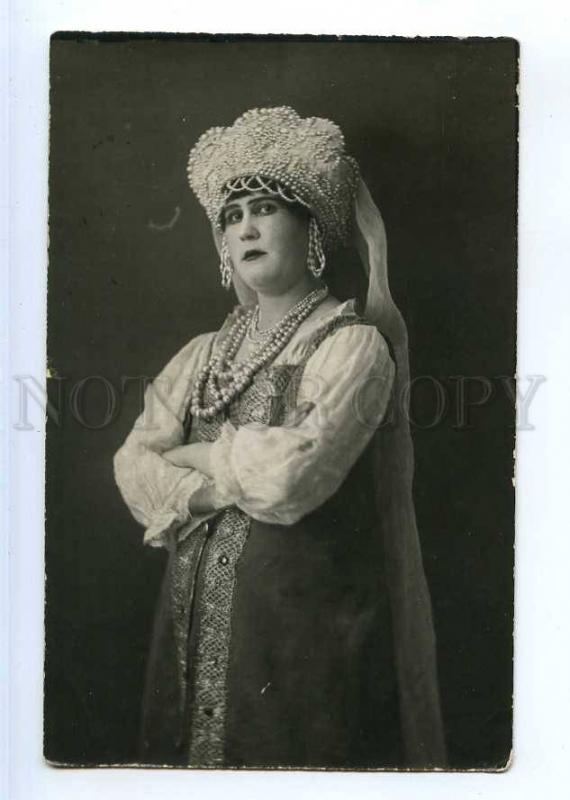This vintage black-and-white photograph, presented in a vertical rectangular format, features a striking portrait of the Russian opera singer Bel Kokoshnik dating back to around 1900. The image showcases an elegantly dressed woman adorned in intricate, traditional attire. She wears a long-sleeved white blouse underneath a dark, brocade vest with elaborate lace details. Complementing her sophisticated ensemble, she sports multiple strands of pearl necklaces and long, teardrop-shaped beaded earrings. 

Her headpiece, an elaborate beaded hat with curved designs, includes a voluminous piece that cascades down her back, resembling a crown but fashioned from material. The photograph's background transitions from dark black at the bottom to a dark gray at the top, bordered by a light blue outer frame. The woman's makeup is pronounced, with heavy lipstick and a slightly frustrated, intense expression on her face. 

Details around her face and the hat reveal a high level of craftsmanship, featuring a long white veil that adds to the traditional and vintage appearance of the image. A watermark across the center reads "not for copy," underscoring its historical and cultural value. The combination of these elements, along with the black-and-white aesthetic, emphasizes the photograph's antique essence and provides a captivating glimpse into early 20th-century fashion and portraiture.